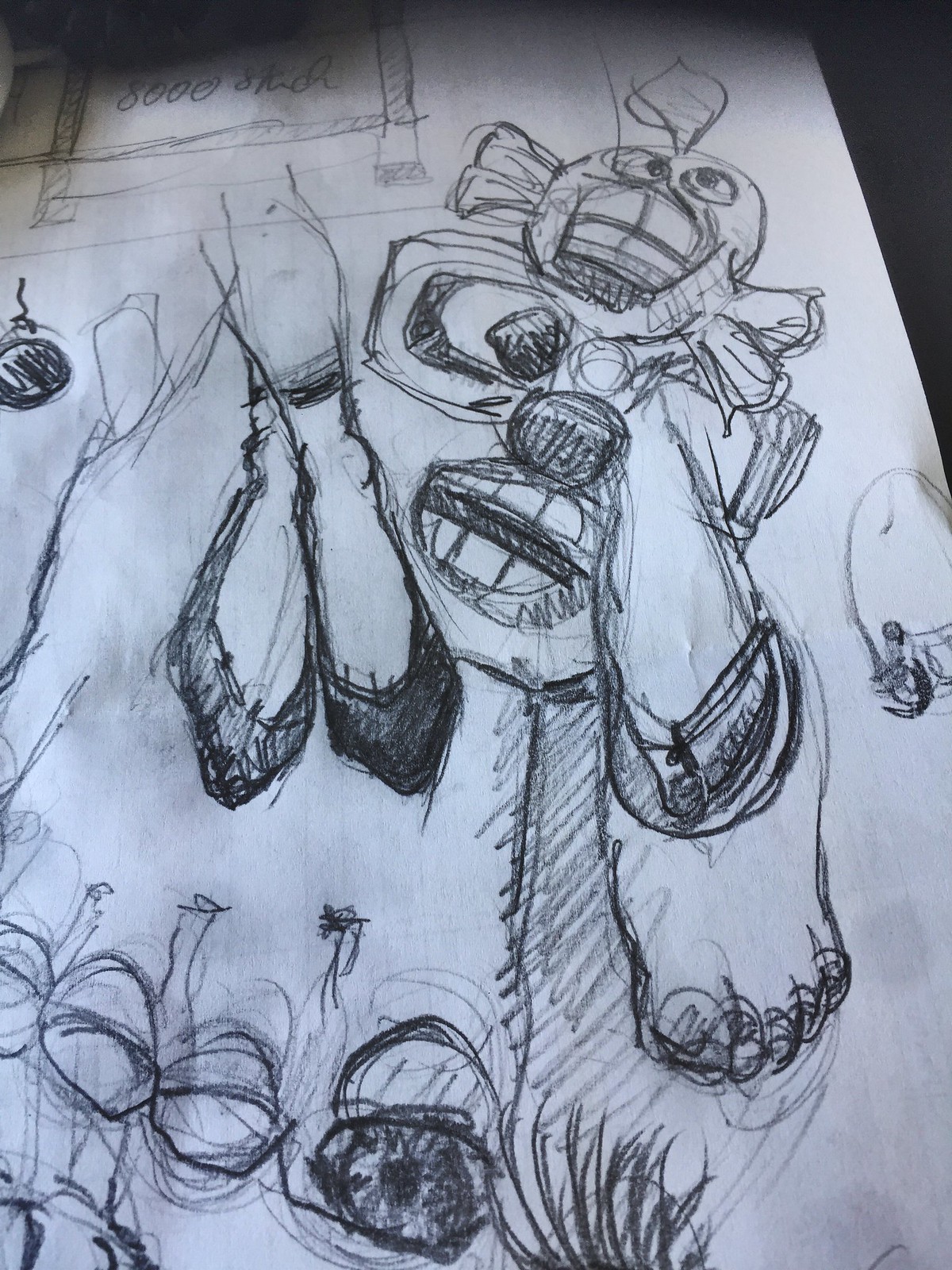This close-up charcoal drawing on white paper primarily focuses on an intricate arrangement of feet and a bear-like face. Dominating the composition is a massive human foot, clearly detailed to show the shape of the toes and the top of the foot. Resting gracefully on top of this large foot are a pair of slender female calves and feet, adorned with darkly colored ballet slippers featuring ankle straps. These feet are crossed delicately, highlighting the contrast against the larger foot beneath them. To the side of these dainty ballet-clad feet, there is a bear's face drawn with striking detail, featuring goggles, a mouth open as if in expression, and brown-colored nose and eyes. From one of the bear's eye sockets, another female foot in flip-flops with painted toenails protrudes and rests on yet another human foot, adding layers of complexity. The feet and face are all meticulously drawn with varying intensities of charcoal, creating a vivid and textured depiction.